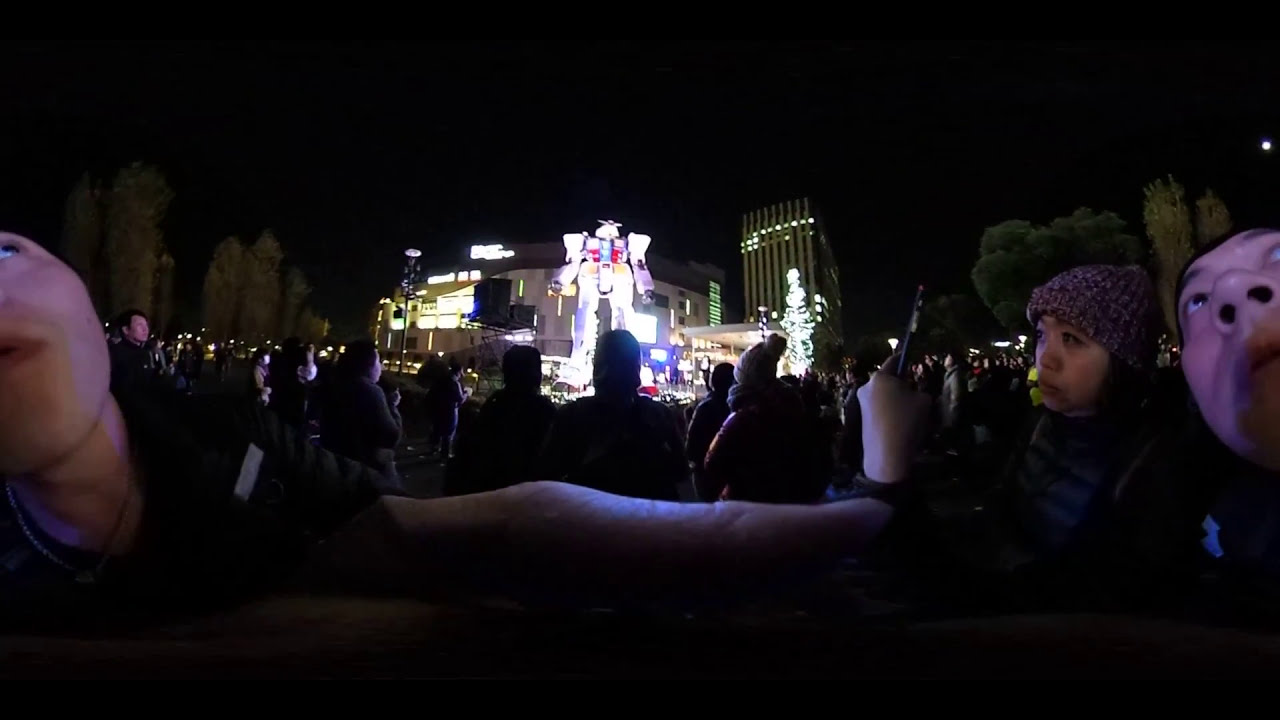This is a photograph taken at night in an urban setting featuring a significant outdoor gathering, likely in Japan. The event appears to center around the unveiling of a giant full-scale Gundam robot, which stands prominently illuminated against a backdrop of skyscrapers and potentially a factory building. The crowd, estimated to range from 100 to 150 people, is depicted from behind, with some individuals turning to face the camera. Notably, a woman wearing a beanie and a man whose upward gaze reveals his nostrils and one eye can be seen on the right, with another person partially visible on the left similarly looking up, possibly at the Gundam. The atmosphere suggests a sense of awe and excitement, as attendees capture selfies and gaze in admiration at the towering, blocky robot that is backlit and about five to six stories tall. The well-lit stage and the ambient city lights add to the festive and bustling nighttime scene.